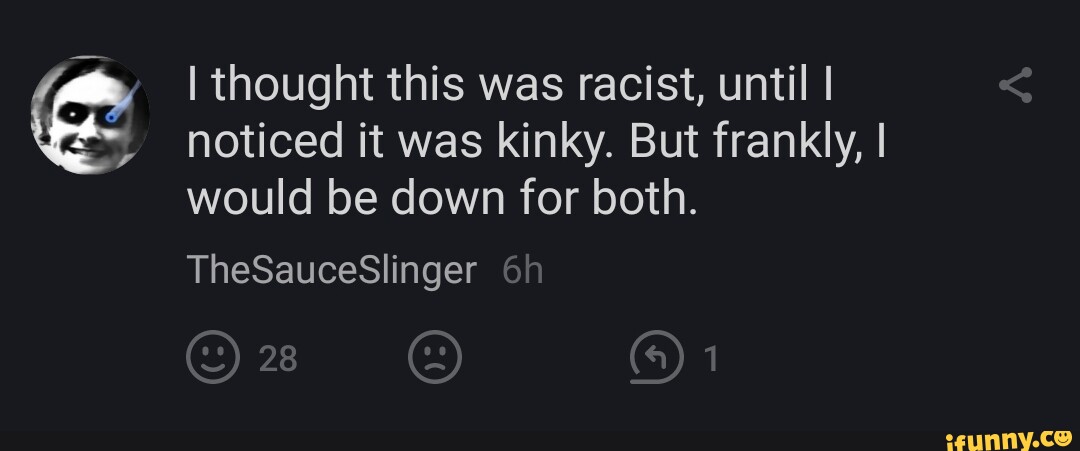This is a rectangular image, probably three times wider than its height, with a black background. In the bottom right corner, in bolded yellow text, it says "ifunny.c," accompanied by a yellow smiley face. In the top left, there's a close-up profile picture of someone with slicked-down black hair. Their eyes have black circles around them, with the left eye depicted as a white dot and the right eye as blue with a small flame coming from the top. The individual has an evil grin.

To the right of the profile picture, in bold white text, the comment reads: "I thought this was racist, until I noticed it was kinky. But frankly, I would be down for both." Below the text, in smaller white letters, it says, "the saucy slinger." To the right in gray text, "6H" indicates the comment's timestamp.

Aligned with the top row on the right side, there's a gray share icon. Below "the saucy slinger," there is a gray outline of a smiley face with "28" next to it, also in gray. Next to that is an outline of a gray frowny face. Further down, there is an incomplete circle icon with an arrow pointing up and to the left, accompanied by a gray "1".

The overall design of the image creates a dark and edgy aesthetic, amplified by the bold contrasts and provocative nature of the comment.